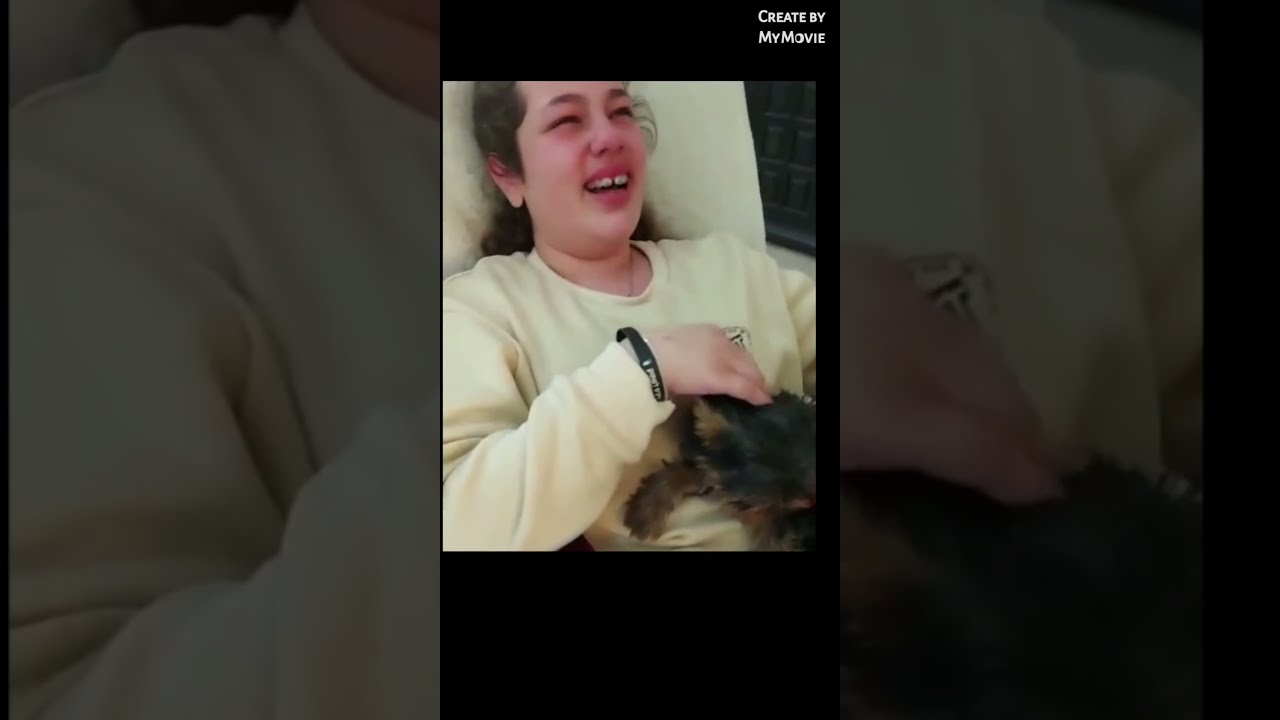The image depicts a young woman with light skin and dark brown hair, which is either tied back or cascading down her back. She is sitting up in bed and leaning against a white pillow. She is laughing heartily, with her mouth open and eyes squinting, revealing a small gap in her front teeth. She has on a white crewneck sweater with a small logo on it, and she wears a black bracelet or watch on her right wrist. Her right elbow rests on a purple and white pillow, which is under her arm. She appears to be holding something furry in her right hand, which might be a small animal, though it is slightly cut off and not clearly visible. The photograph is part of a triptych, with the central image flanked by two close-up columns: the left column focuses on her right arm and the pillow, while the right column highlights her right wrist and bracelet. The top right corner of the image has a caption in white letters that says, "Created by My Movie." The overall composition has a black border on the top third and right side, giving it a framed effect.